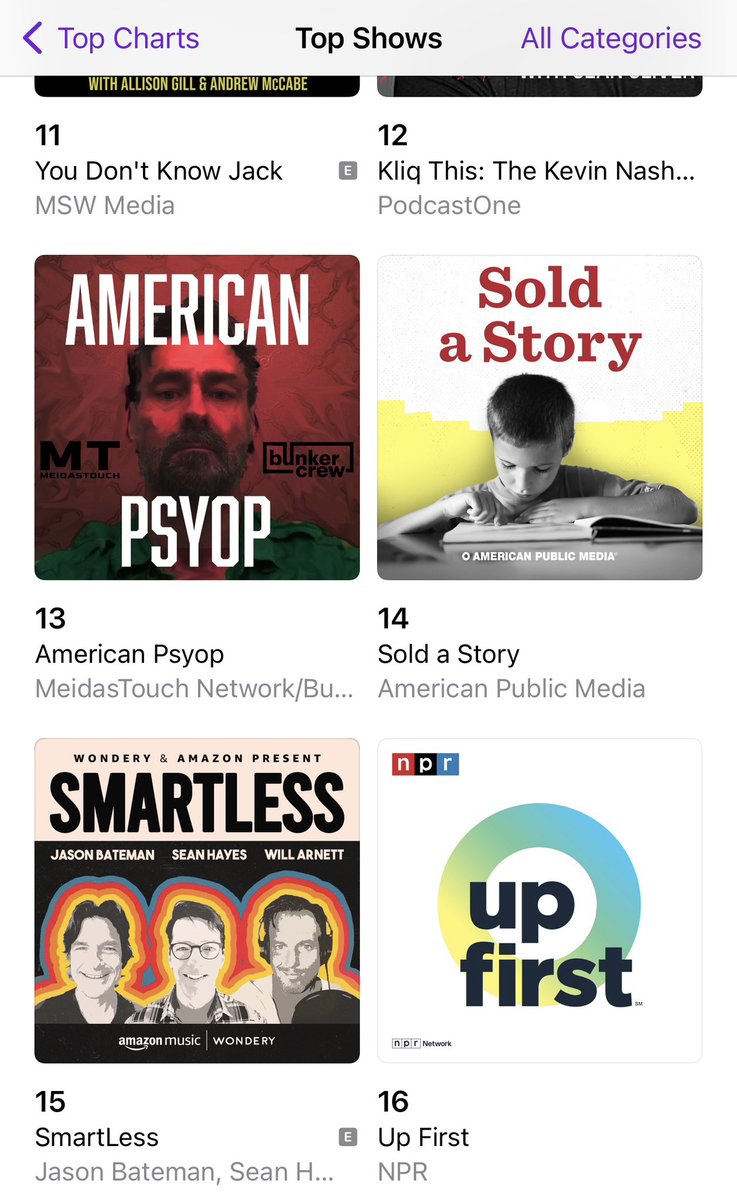The image showcases a list of top TV shows, highlighted under the heading "Top Shows in Black" at the top of the page. On the right side, there's a purple button labeled “All Categories,” while on the left side, it reads "Top Charts," also in purple, akin to the back button placed nearby. Centered on the page is a white background featuring the ranked TV shows from numbers 11 to 16.

At the top right corner, the number 11 entry is “Who Don’t Know Jack” by MSW Media. This show features an icon themed "American Psyop Media MT Banga Crew," set against a red and green background with a picture of a man. Moving down, the number 12 entry is also prominent at the top right, with an interactive click option suggesting further details. 

Following the ranks:
- Number 13 is “American Psyop” by Media Search Network.
- Number 14 is “Solve a Story” by American Public Media.
- Number 15 is “SmartLess” by Jason Pettiman.
- Number 16 is “Up First” by NPR. 

The layout and details of each show are meticulously organized to provide an informative glance at the rankings and associated media.